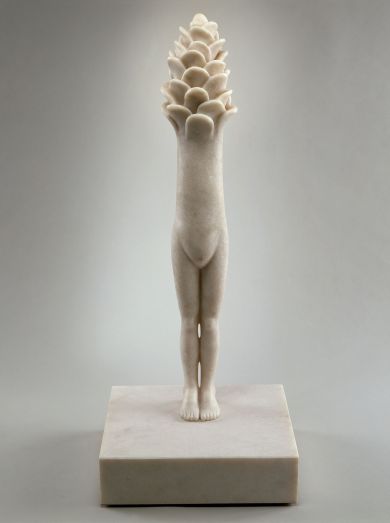The image features a detailed and intriguing sculpture prominently positioned in the center of an off-white background. It rests on a square base, potentially crafted from white marble or alabaster. The sculpture itself combines the form of a human and an organic element, creating a striking visual. 

From the base, the sculpture begins with a nude human figure depicting two feet and legs up to the waist, complete with defined anatomical details like a belly button. The legs are closely positioned with a slight gap near the knees and lower ankles that allows light to pass through. The human element is rendered in a monochromatic scheme of gray, off-white, and subtle black hues.

As the sculpture progresses upwards from the waist, the human form transforms into a series of layered petals resembling an artichoke or possibly a blooming flower, rising to where the neck and head would typically reside. The petals are intricately crafted, with approximately six layers clearly visible, creating a harmonious blend between human anatomy and botanical elements.

This unique and thought-provoking artwork, lacking text or identifying information, evokes a sense of curiosity and could easily be an exhibit in a museum. The absence of external features, such as arms or a head, and the transformation into vegetal petals, endows the sculpture with an enigmatic and artistic allure.